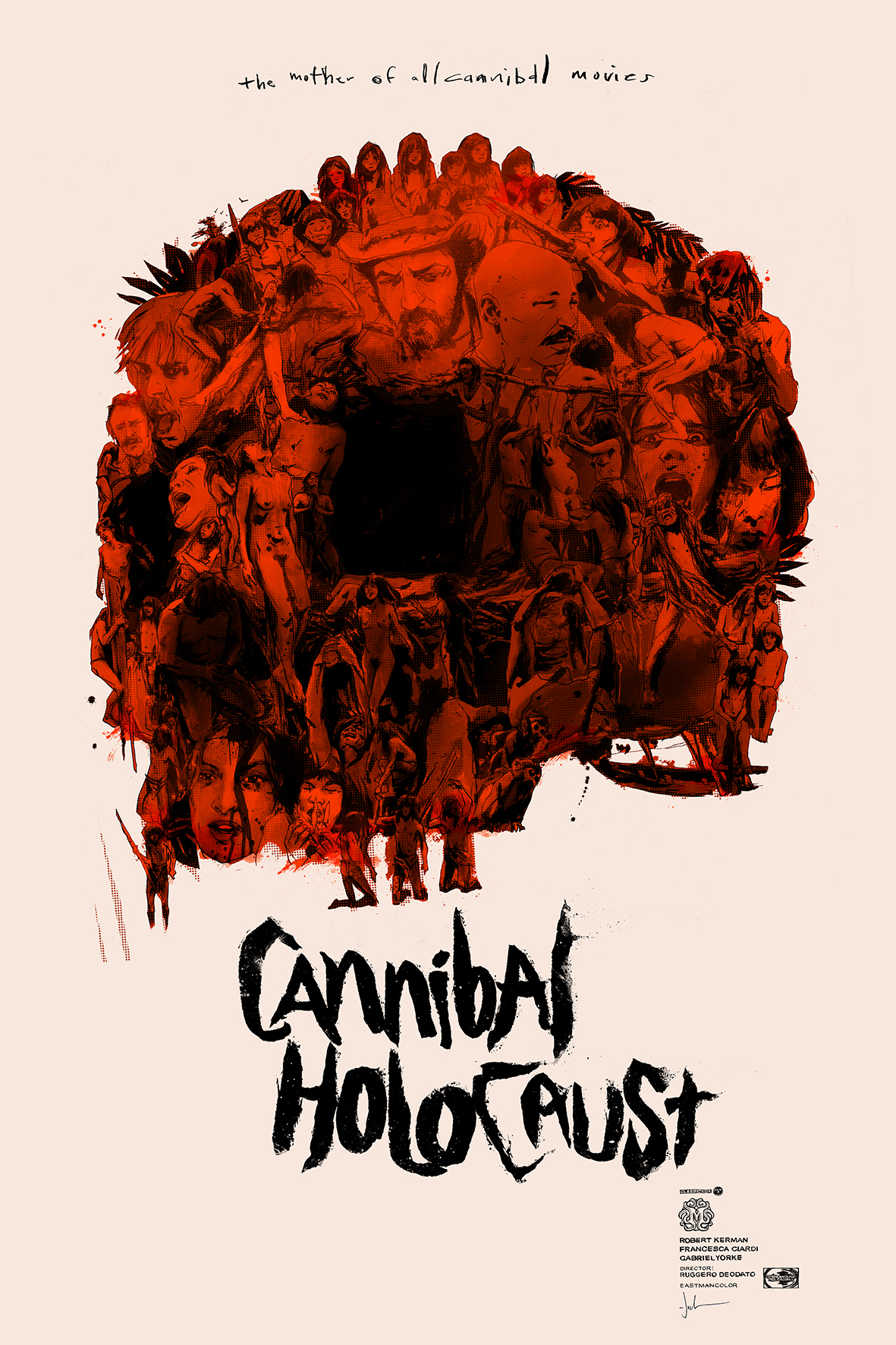This is an image of a movie poster with a beige or pinkish background, featuring a striking visual collage as its centerpiece. Dominating the poster is an artistic, circular arrangement of faces drawn in red and black, resembling a skull. The faces throughout the collage appear grotesque and distressed, evoking a sense of horror and chaos. At the very top, in a messy, handwritten style and small font, is the phrase "The mother of all cannibal movies." Below this macabre circle, the title "Cannibal Holocaust" is prominently displayed in a large, stylistic font that looks hand-drawn with broad strokes. Within the circular collage, details include three people standing at the bottom center, one person on the bottom left holding what seems to be a sword, a woman's face also at the bottom left, and a man with a hat at the top. A black hole in the middle of the circle adds an unsettling void to the composition. The bottom right corner of the poster contains small, unreadable text and an indistinct emblem or design.